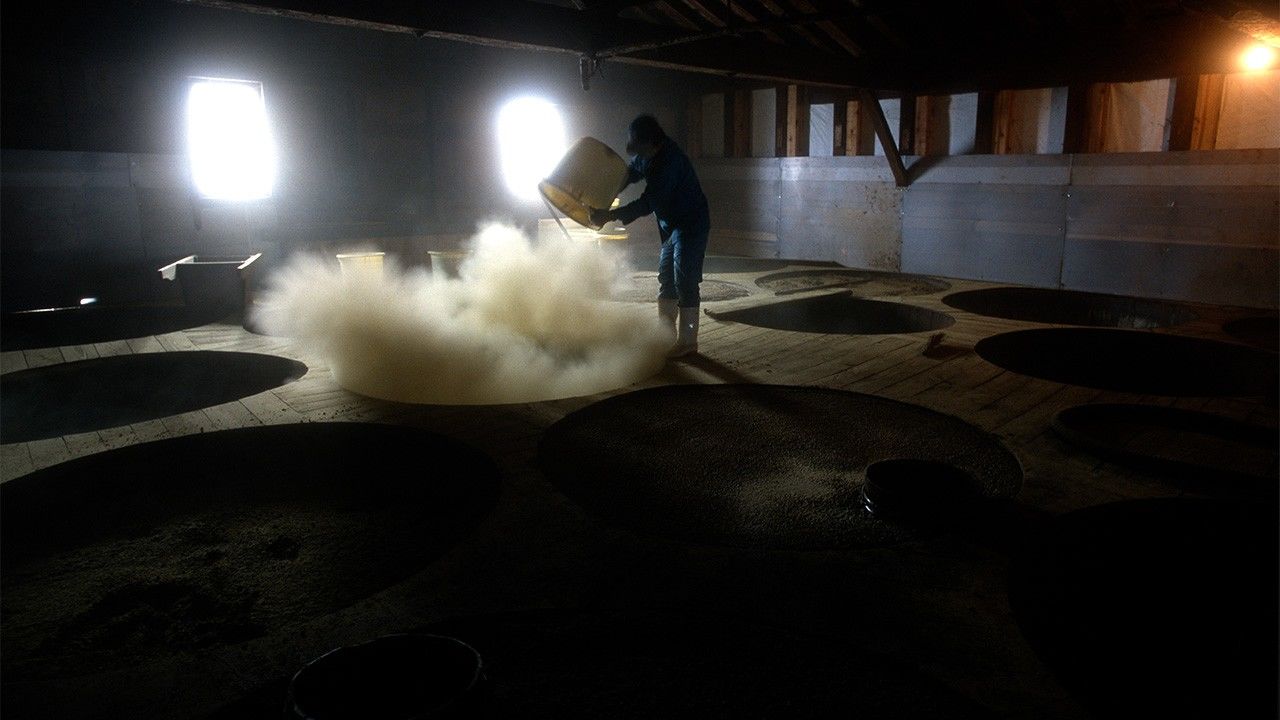The image depicts a very dimly lit, basement-like warehouse with a combination of two white lights and one yellow light providing minimal illumination. The dark, cement structure features a wooden floor riddled with numerous holes. In the foreground, a man is engaged in manual labor, holding a yellow bucket from which he has just poured an unknown liquid into one of the floor holes. This action has caused a cloud of dust and steam to rise into the air, adding to the murky atmosphere. The room's brick walls and wooden support beams are faintly visible under the sparse lighting, and four more buckets are seen in the background, suggesting that the man has additional tasks to complete.